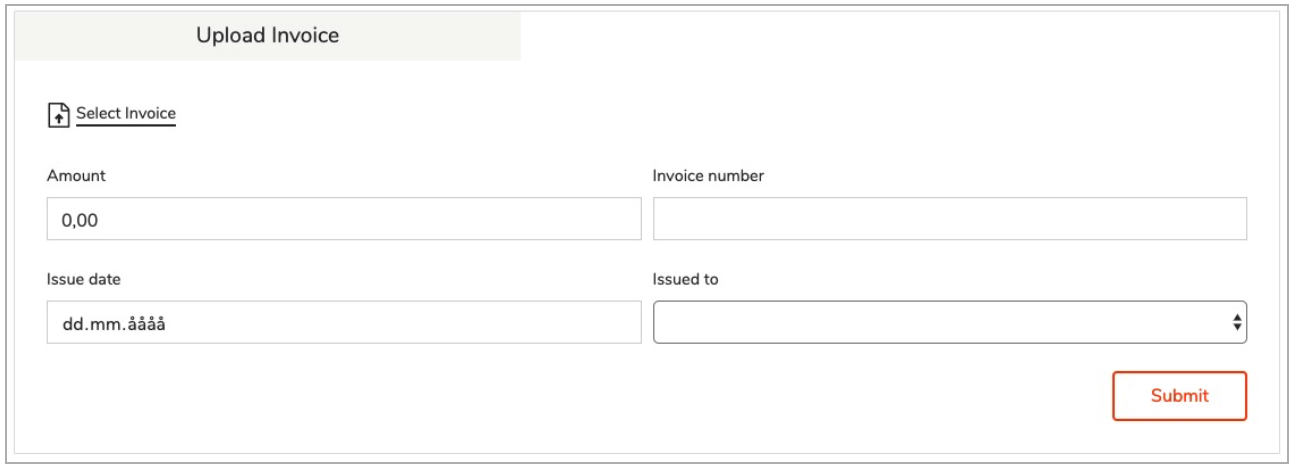The image portrays a blank invoice form designed for online entry. At the top of the form, the header reads "Upload Invoice" with a subtle gray shading beneath it, which distinguishes it from the rest of the form. Below this, there is a button labeled "Select Invoice."

The form includes several fields for data entry:

- **Amount:** A field pre-filled with "0.00" where an amount can be entered.
- **Invoice Number:** This field is currently blank.
- **Issue Date:** Placeholder text "dd.mm.yyyy" is present, indicating the required date format.
- **Issue To:** This field is also blank and has a caret icon on the right side, suggesting a dropdown menu or a selection option.

At the bottom of the form, there is a prominent "Submit" button, featuring red text on a white background, encased in a red outline.

The overall design of the form is clean and minimal, primarily utilizing white space and black font, with a horizontally oriented rectangular layout. This form is likely intended to be filled out and then uploaded to a client through some sort of digital platform, although no specific website or additional context is provided in the image.